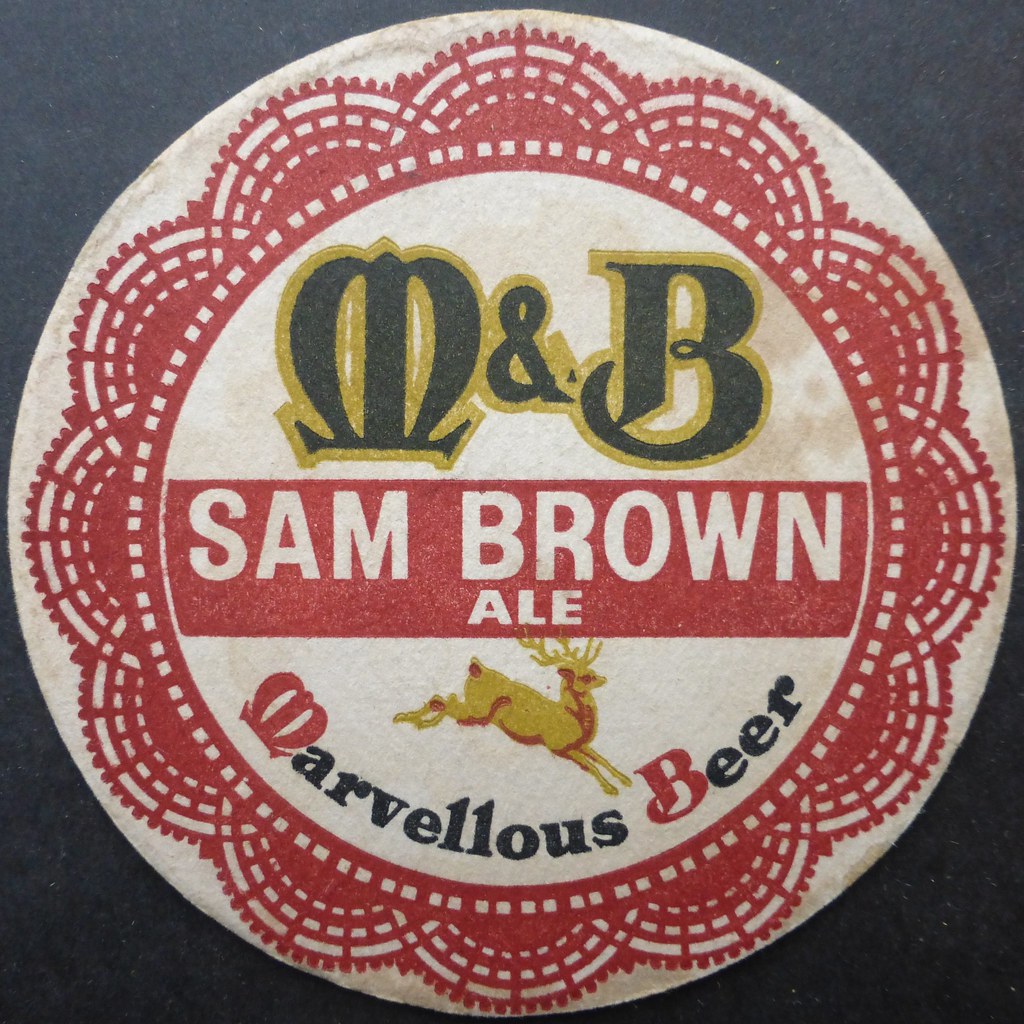A captivating beer pin set against a dark gray background, featuring intricate design elements. The centerpiece is a slightly stained white circle. Within this circle resides a striking red sunburst design, punctuated by cut-out squares that reveal the white backdrop beneath, forming an engaging play of colors. Central to the design is another white circle housing green text with a shadow effect that reads "M&B" at the top. Directly below the text, a prominent red rectangle contains the label "Sam Brown Ale" in bold white lettering. Adding an artistic touch, a golden-hued deer is dynamically illustrated below, its antlers extending up into the red rectangle. The deer appears in motion, its legs gracefully posed as if bounding forward. Completing the design, a semicircular inscription at the bottom reads "Marvelous Beer," with the "M" and "B" highlighted in red and the remaining text in elegant black.